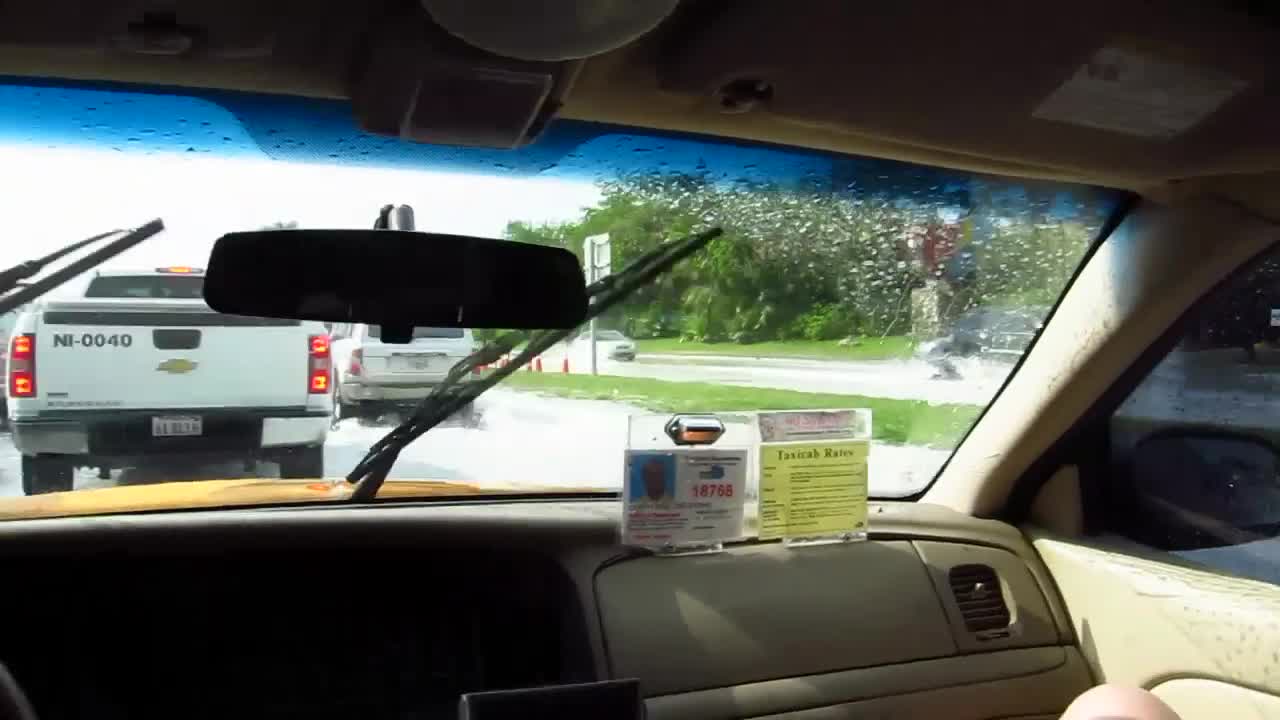This daytime photograph captures a rainy scene from inside a vehicle, possibly a taxi. The windshield is wet, and the windshield wipers are in motion, indicating active rainfall. The view through the windshield reveals a multi-lane road with a truck and an SUV directly ahead of the vehicle. A strip of grass separates the lanes of traffic, and thick, lush green trees line the side of the road. The dashboard is visible in the foreground, with the rearview mirror in sight. On the passenger side, a taxi cab rate sign is mounted above the glove box, accompanied by additional text. To the left, a photograph of the driver and his taxi license number are clearly displayed, suggesting this is indeed a taxi.